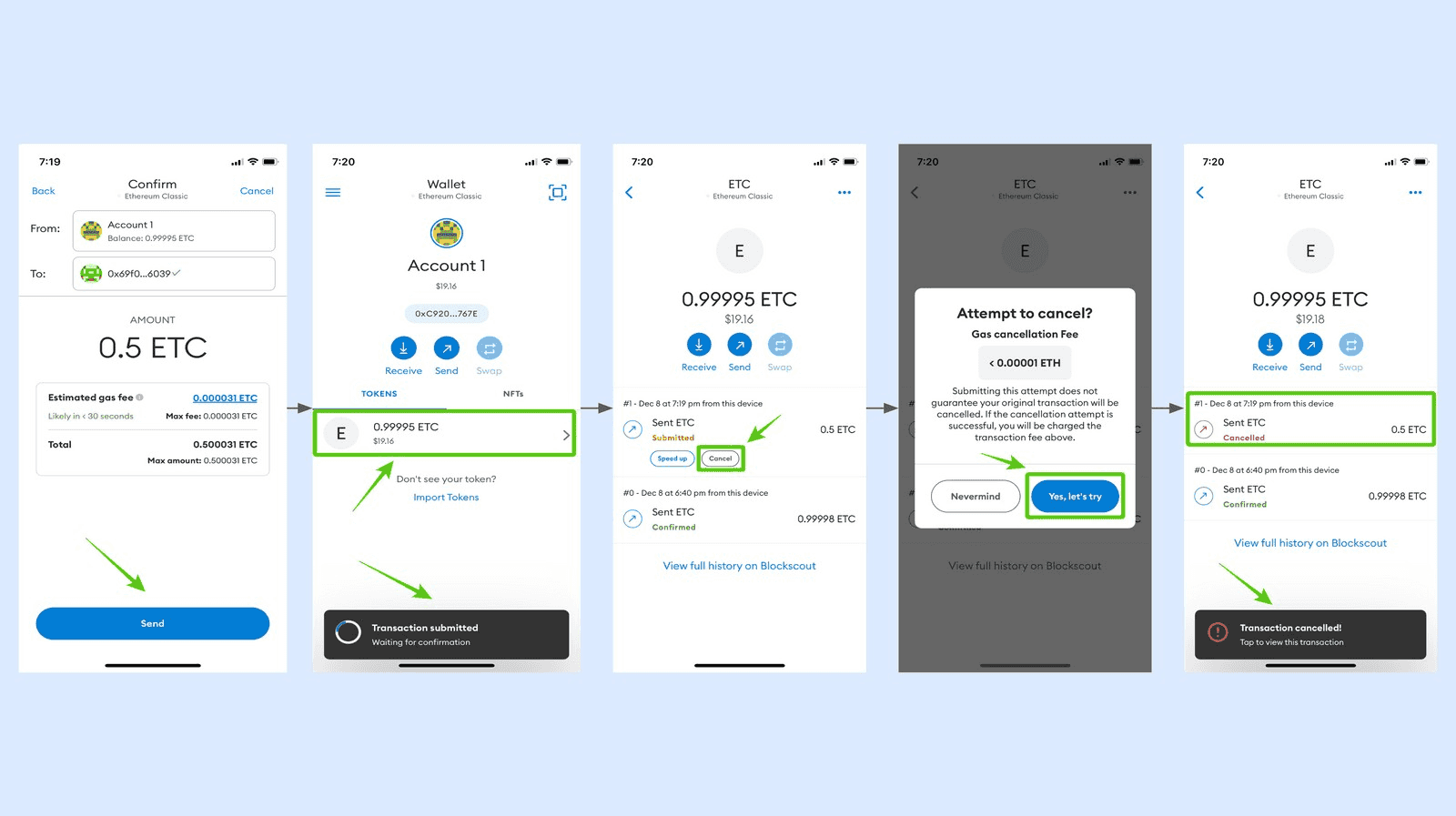The image features a light blue background with five separate screenshots of a mobile device or tablet screen, as indicated by the visible battery symbol, Wi-Fi icon, and time display in the upper left corner, mostly showing 7:20, except for the first screen which shows 7:19. These screenshots display an application with a predominantly white interface, black text, and blue buttons. 

1. The first screenshot shows a confirmation screen for an ETC (Ethereum Classic) transaction. It details "Account 1" sending 0.5 ETC to another account, including an estimated gas fee and a total of 0.5 ETC. A blue button with a green arrow is visible.
  
2. The second screenshot features "Account 1" with options to "Receive" and "Send" ETC, displaying the account balance. A notification bubble at the bottom reads "Transaction Submitted."

3. The third screenshot displays the ETC wallet page showing a balance of 0.999 ETC, equivalent to $19.16. It includes "Receive," "Send," and a highlighted "Cancel" button.

4. The fourth screenshot presents an "Attempt to Cancel" window with information on the gas cancellation fee. A blue button labeled “Yes, Let’s Try,” highlighted in green, is shown.

5. The fifth screenshot again shows the ETC wallet page, with options to "Receive" and "Send." It highlights a "Sent ETC" transaction that has been canceled, along with a notification bubble stating "Transaction Canceled."

These images collectively demonstrate how to use the app to send, receive, and cancel Ethereum Classic transactions.